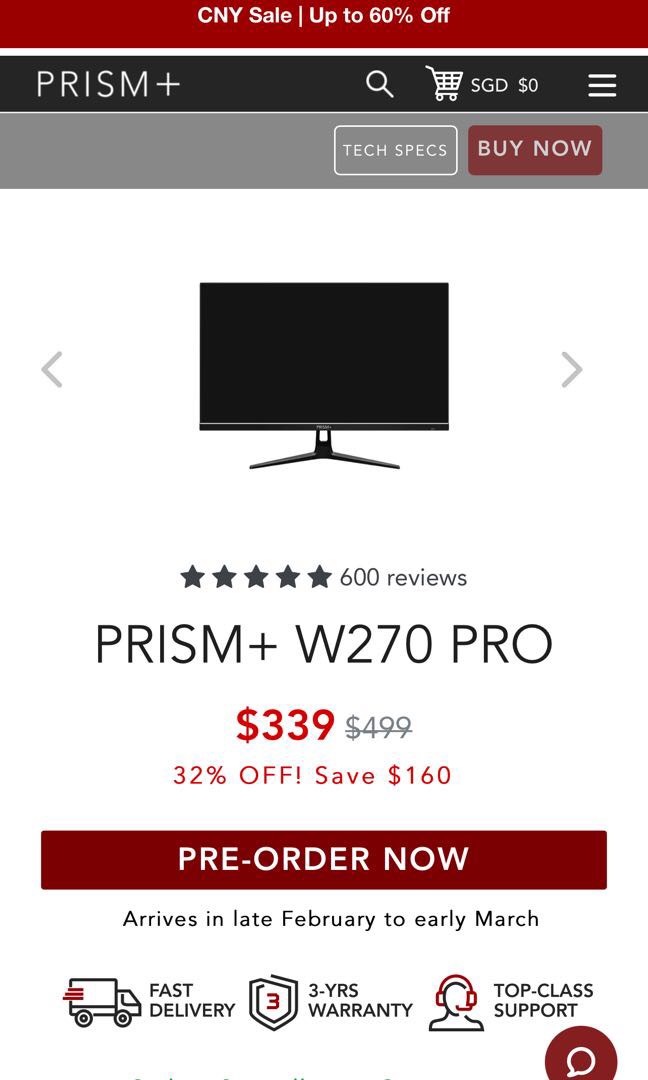**Detailed Advertisement Description:**

At the top of the image, a bold red banner hosts an advertisement, featuring prominent white text that reads, "CNY Sale - Up to 60% Off." Below this, the design elements include sleek black text showing "Prism+," a magnifying glass icon, a shopping cart icon, and the currency abbreviation "SGD" in two instances, followed by a dollar sign and "03." White lines are neatly aligned above a gray line that separates these details from the main promotional content.

In the central part of the image, a well-defined black TV screen stands out, adorned with gray arrows pointing left and right. Directly beneath it, there are five stars in a brown or gray color, indicating a rating alongside "600 reviews.”

Further down, the product name "Prism+ W270 Pro" is clearly displayed. The current price of "$339" is highlighted in red, with the original price "$499" in gray, crossed out to show a significant discount. Above a red box, "32% off – Save $160" is in vibrant red text. The red box itself features a call-to-action in white font, "Pre-Order Now." Below, gray text promises that the product will arrive between late February to early March, accompanied by a truck icon and the text "Fast Delivery."

Adjacent to the main product information, a series of icons and brief descriptions provide additional selling points. One icon features a red "3" surrounded by a shield outlined in gray, signifying, "3 Years Warranty." Another icon depicts a person wearing red headphones, labeled "Top-Class Support." Lastly, a reddish-brown circle with a white center completes the detailed advertisement.

This extensive imagery is designed to attract customers by providing a comprehensive breakdown of the offer, product highlights, and value-added services.